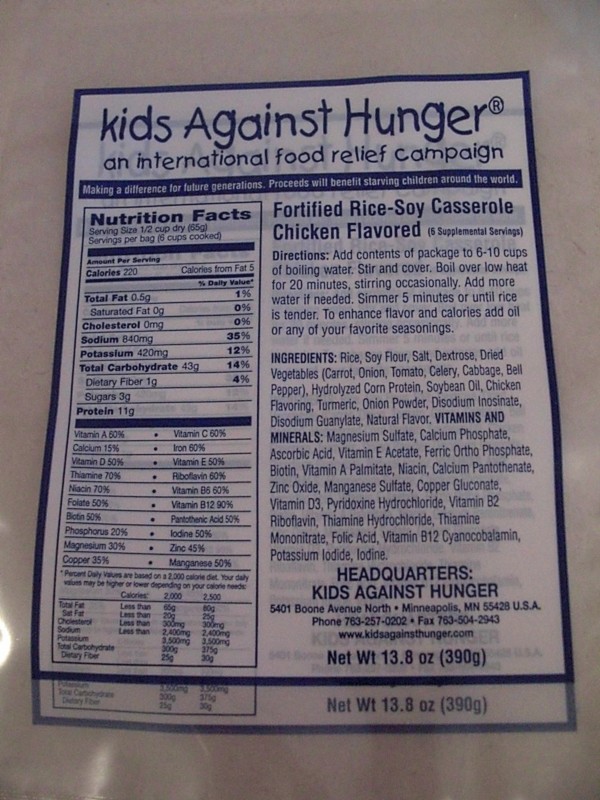This photograph captures the back label of a food package for a fortified rice soy casserole with chicken flavor. The label prominently features the Kids Against Hunger logo, an international food relief campaign dedicated to combating hunger. Detailed nutrition facts are provided in an easy-to-read panel, ensuring consumers are well-informed about their dietary intake. A comprehensive list of preparation directions guides users through the cooking process, while another section meticulously outlines the ingredients used in the product. Additional information about the Kids Against Hunger headquarters is also included, emphasizing the organization's commitment to global food relief. The net weight of the package is specified as 13.8 ounces (390 grams), with each serving size equating to one half cup of the dry mix.